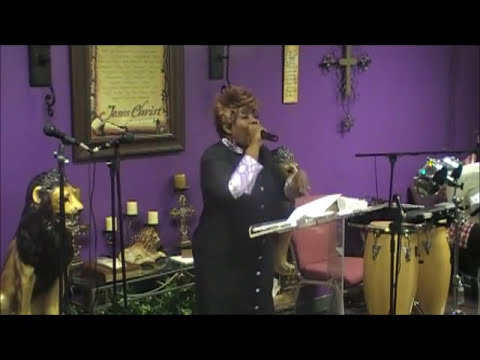The image captures a black woman with short, light brown hair standing in an African church, likely in the midst of singing or speaking. She is wearing a dark-colored dress with buttons down the front and a white shirt underneath. With her right hand, she holds a microphone up to her mouth and stands behind a clear podium meant for holding music. Her eyes are closed, adding an air of concentration or emotion to the moment. The setting features a bright purple wall adorned with several items, including a large crucifix, a framed document with cursive text reading "Jesus Christ," and another wall hanging with inscriptions. To her left, there's a table bedecked with candlesticks, additional microphones on stands, and a ceramic lion figure. To her right, the image shows bongo drums, possibly accompanied by a snare drum, with some flowers visible in the background. Black borders frame the top and bottom of the photograph.